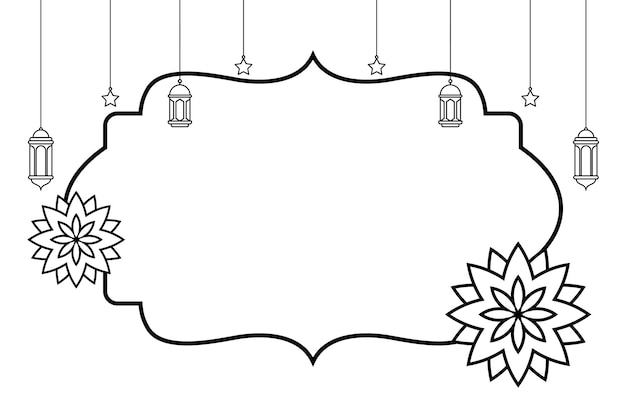This digital black-and-white illustration features a central, bubble-like shape with jagged, pointed outlines, giving it a resemblance to a thought bubble. Inside this ambiguous shape, the background remains plain white. On the lower left and right sides of this bubble, there are intricately designed geometric flowers. Each flower is built with triangular tips and layers, culminating in a six-petaled star shape at the center with a tiny black core. The flower on the right appears larger than its counterpart on the left, bringing a sense of balance to the design.

Suspended from thin vertical lines at the top of the illustration are a total of eight elements, alternating between lanterns and small stars. These lines vary in length, with the longest ones extending from the upper left and right corners. The lanterns and stars hang in an elegant, interspersed pattern, contributing to the intricate and sophisticated feel of the artwork. The delicate interplay between the hanging elements and the central bubble-like shape combines to create a visually engaging and thoughtfully composed image.